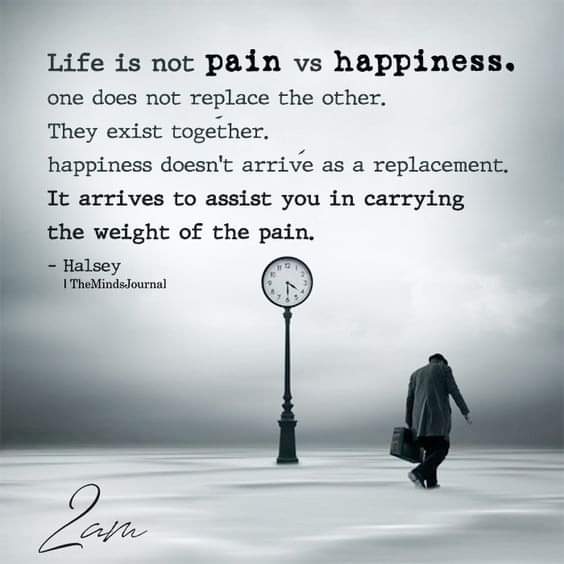The image is a large square motivational graphic primarily in black, white, and various shades of gray. The background features a thick, overcast sky that melds into a foggy, desolate ground, giving a sandy, uneven appearance. Central to the scene is an old-fashioned street clock atop a black metal pole, displaying the time as 4:30. Walking away from the viewer towards the right, a man in a dark gray coat, black pants, and a black hat carries a suitcase in his left hand, looking downward as he moves through the bleak setting. The inspirational text at the top of the image is left-aligned and says, "Life is not pain versus happiness. One does not replace the other. They exist together. Happiness doesn't arrive as a replacement. It arrives to assist you in carrying the weight of the pain." The words “pain” and “happiness” are bolded for emphasis. The quote is attributed to Halsey and appears in the Minds Journal. In the bottom left-hand corner, there is an indistinct cursive signature, possibly reading "Z A N U." The overall imagery and message suggest a theme of resilience and coexistence of emotions, ideal for sharing on social media or a personal blog.